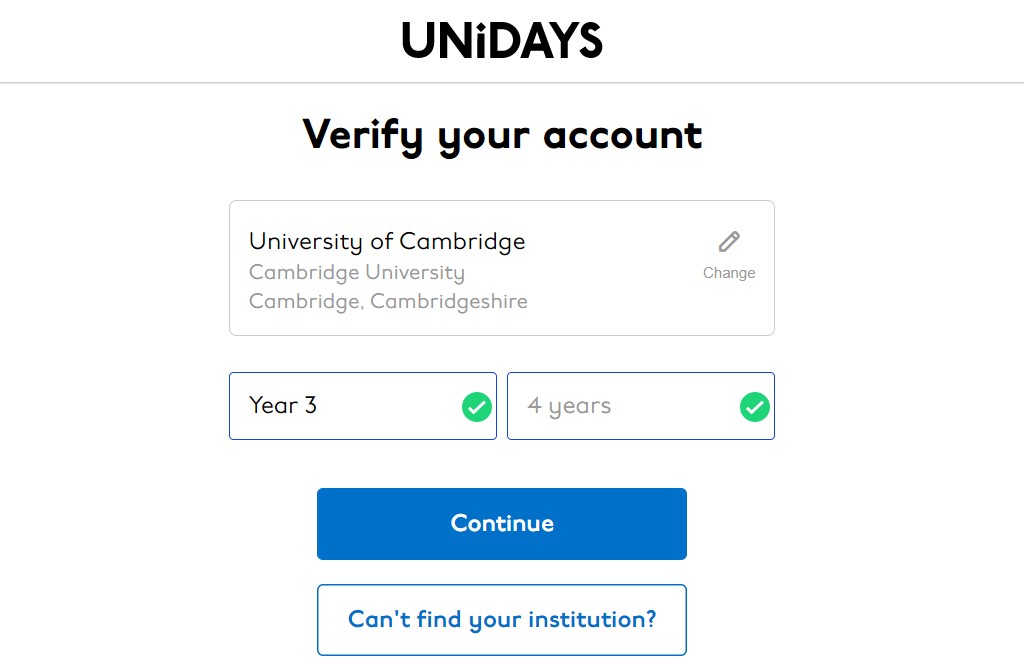The image showcases the Unidays website interface. At the top center of the screen, the site's name "unidays" is displayed in a lowercase black font. Directly below this is a thin grey line extending across the width of the screen. Beneath the line, a black-font title reads "Verify Your Account." 

Following the title is a grey rectangular box with a bold, black heading inside it that states "University of Cambridge." Below this heading, in grey text, are the words "Cambridge University, Cambridge, Cambridgeshire." On the right side of this information is a pencil icon accompanied by the word "Change," which allows users to edit these details if necessary. 

Below this section is a dark grey edit box containing the text "year three" on the left side, paired with a green circle featuring a white tick on the right side. Adjacent to this is another edit box with the value "four years" in light grey text, also accompanied by a green circle with a white tick. 

At the bottom of the screen, there is a prominent blue button labeled "Continue," followed by a secondary white button with blue text that reads "Can't find your institution."